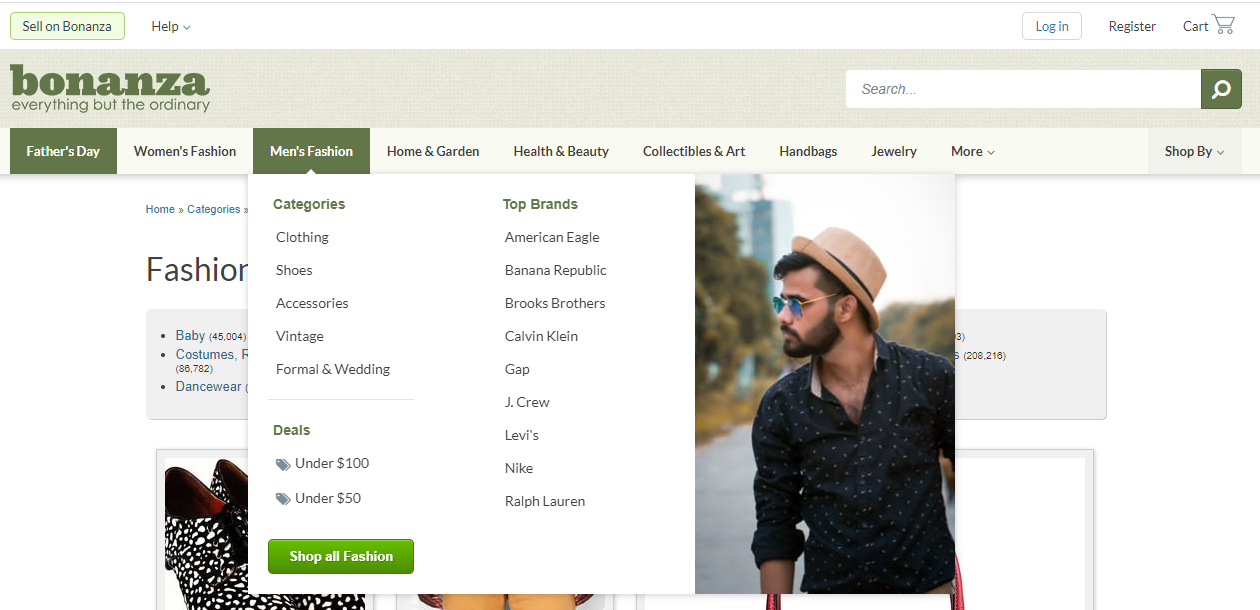A detailed website screenshot caption:

"In this screenshot of the Bonanza website, the top-left corner prominently features the Bonanza name in dark green text, complemented by the tagline 'Everything but the ordinary' in smaller, lighter green text beneath it. Just above the logo, there's a prominent green button labeled 'Sell on Bonanza' and to its right, a 'Help' button with a drop-down menu symbol. Directly below the logo is the website's navigation bar with several tabs: 'Father's Day,' indicating that the screenshot was likely taken in early to mid-June, 'Women's Fashion,' 'Men's Fashion,' 'Home and Garden,' 'Health and Beauty,' 'Collectibles and Art,' 'Handbags,' 'Jewelry,' and a 'More' tab.

On the top right of the navigation bar, there's a 'Shop by' option with a drop-down arrow. The cursor or selection is currently on the 'Men's Fashion' tab, revealing a drop-down menu with subcategories including 'Clothing,' 'Shoes,' 'Accessories,' 'Vintage,' 'Formal,' and 'Wedding.' To the right of these subcategories, there's a list of top brands featuring names such as American Eagle, Banana Republic, Brooks Brothers, Calvin Klein, Gap, J.Crew, Levi's, Nike, and Ralph Lauren."